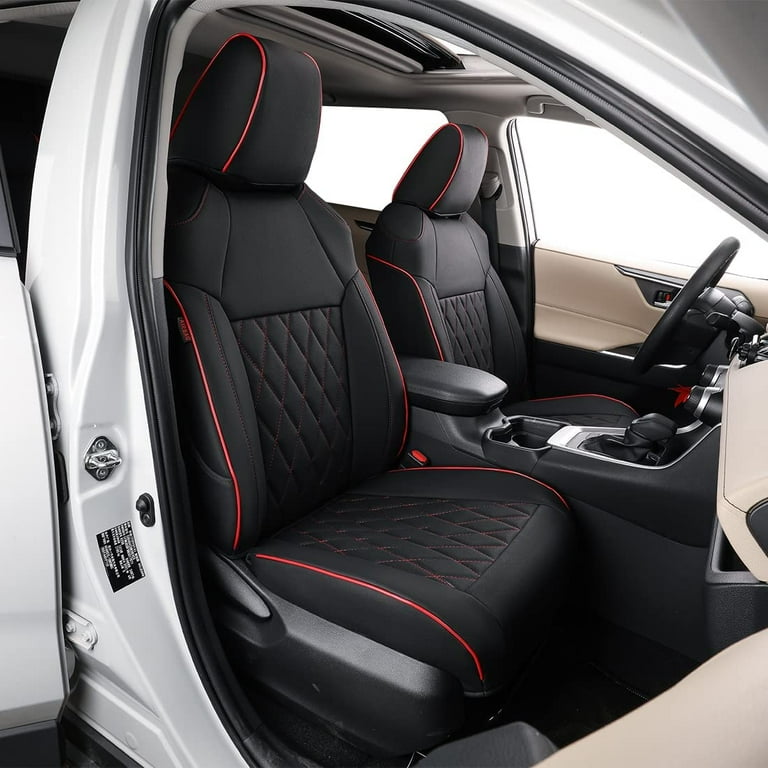This image captures the interior of a white vehicle, likely a pickup or an SUV, with an open passenger-side door and a visible front section. The interior exudes a pristine and new appearance, featuring black high-back bucket seats accented with red trim around the edges and tufted upholstery on the seating area. The seats are detailed with a quilted pattern on the backrest. The interior color scheme includes a combination of tan, black, and grey tones. The front console has a tan-cream color while the area around the center console, which houses the gearshift, exhibits grey and black accents. The doors, both the rear and front door on the passenger side, are open, providing a clear view of the clean and neatly arranged cabin. The inside panel of the door is predominantly white with grey elements, completing the sophisticated and uncluttered look of this well-maintained vehicle.